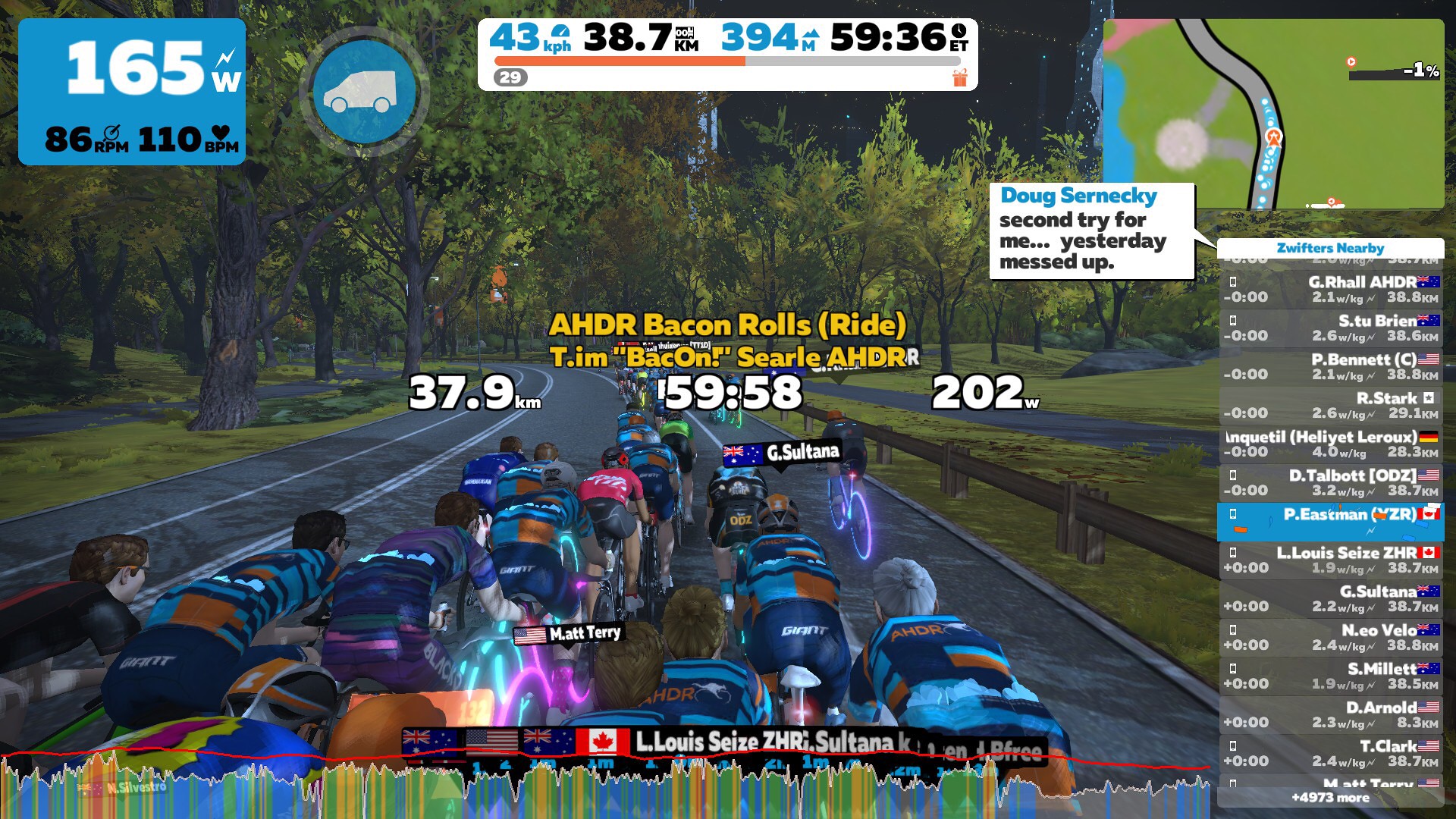The image is a screenshot from a cycling video game, likely Zwift, showcasing a bike race. At the center, a group of digitally rendered bicyclists in uniforms are seen riding along a curving trail lined with large oak trees bearing yellow leaves and a brown barrier on the right side to prevent them from veering off the track. There are about 20 bicyclists, all appearing bent over their bikes, seemingly in intense competition. At the bottom of the screen, various country flags, including the UK, US, and Canada, are visible, with the main text focusing on a rider named L. Lewis, suggesting this player may be in the lead. Player names and other information are displayed alongside the flags. The right side features a list titled "Zwifters Nearby," showing the names of other participants. Additional details include multiple data boxes: the top left box displaying metrics like 165W, 86RPM, and 110BPM, and another blue square showing a truck logo. The top of the screen has a white banner with numbers and letters such as 43KPH, 38.7RM, 394M, and 5936ET, displaying various race statistics. The center portion has additional text, mentioning events like "HDR bacon rolls ride" and specific metrics, ensuring a detailed, immersive gameplay experience.